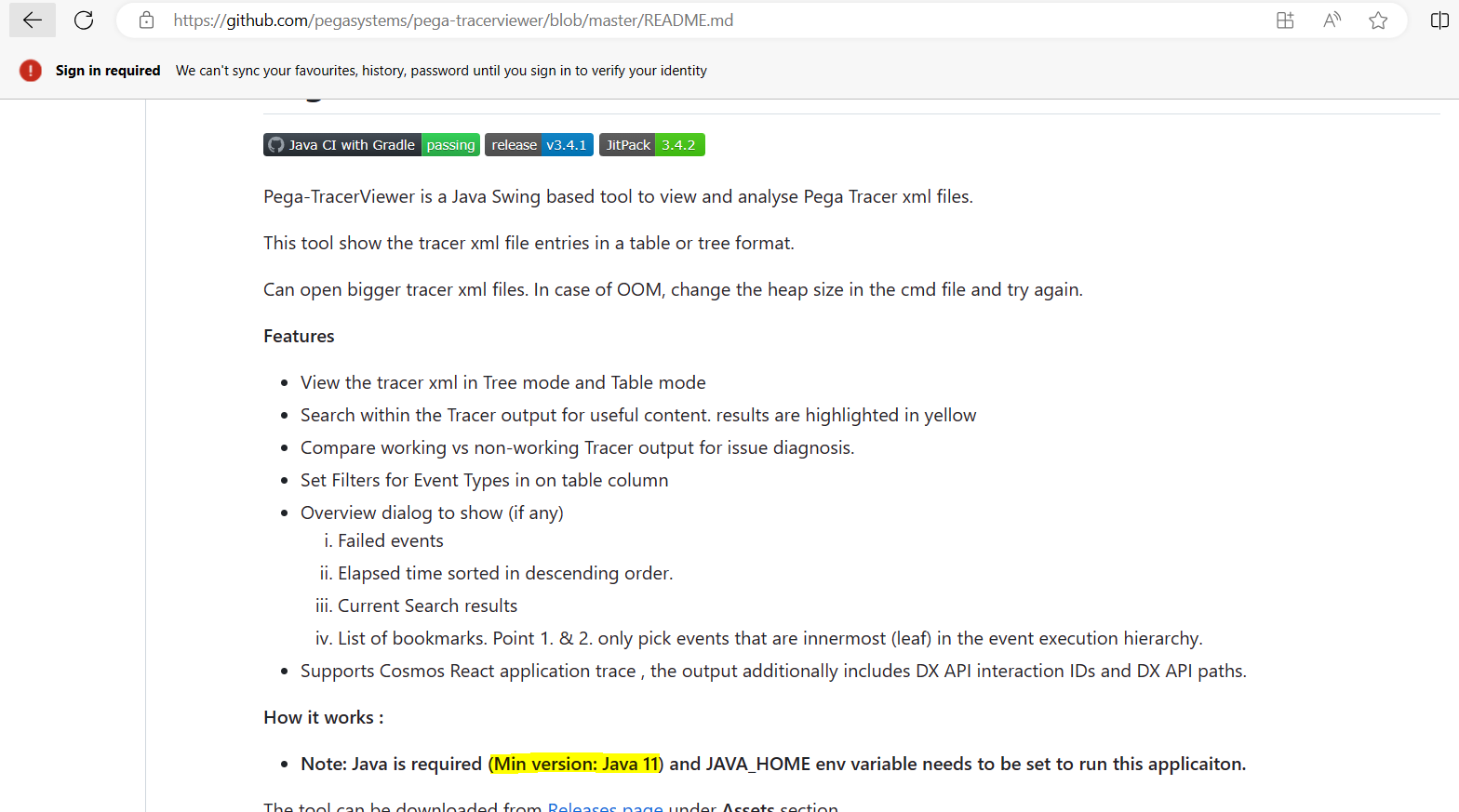**Detailed Caption:**

The image is a screenshot from the GitHub website, specifically featuring the repository page for "Pegasys Systems - Pega Tracer Viewer." The address bar clearly displays "github.com," confirming the website’s origin. At the top of the page, there is a notification overlay with a red exclamation mark indicating that sign-in is required. The message reads, "We can't sync your favorites, histories, and passwords until you sign in and verify your identity."

In the primary section of the screenshot, the repository details are displayed. The page mentions "Java CI with Gradle" and indicates a passing build for release version 3.4.1, further elaborated as "JIT Pack 3.42." Below that, a description of the "Pega Tracer Viewer" is provided. It is explained as a Java Swing-based tool designed to view and analyze Pega tracer XML files, presenting entries in either a table or tree format. The tool offers functionality to open larger tracer XML files and provides guidance to adjust heap size via the CMD file if an Out Of Memory (OOM) error occurs.

Key features of the tool are highlighted, including:
- Viewing tracer in XML tree or table mode.
- Searching within the tracer output, with results highlighted in yellow.
- Comparing working versus non-working tracer outputs for issue diagnosis.
- Setting filters for event types in the table column.
- An overview dialog that presents failed events, elapsed time sorted in descending order, current search results, or a list of bookmarks.

The page also provides a brief "how it works" section, emphasizing that Java is required to run the application, with a minimum version of Java 11 and a properly set JAVA_HOME environment variable. Notably, the "Minimum version Java 11" is highlighted in yellow for emphasis.

Lastly, there is a mention that the tool can be downloaded from the release page, under what appears to be the "assets" section, though this part of the screenshot is partially cut off.